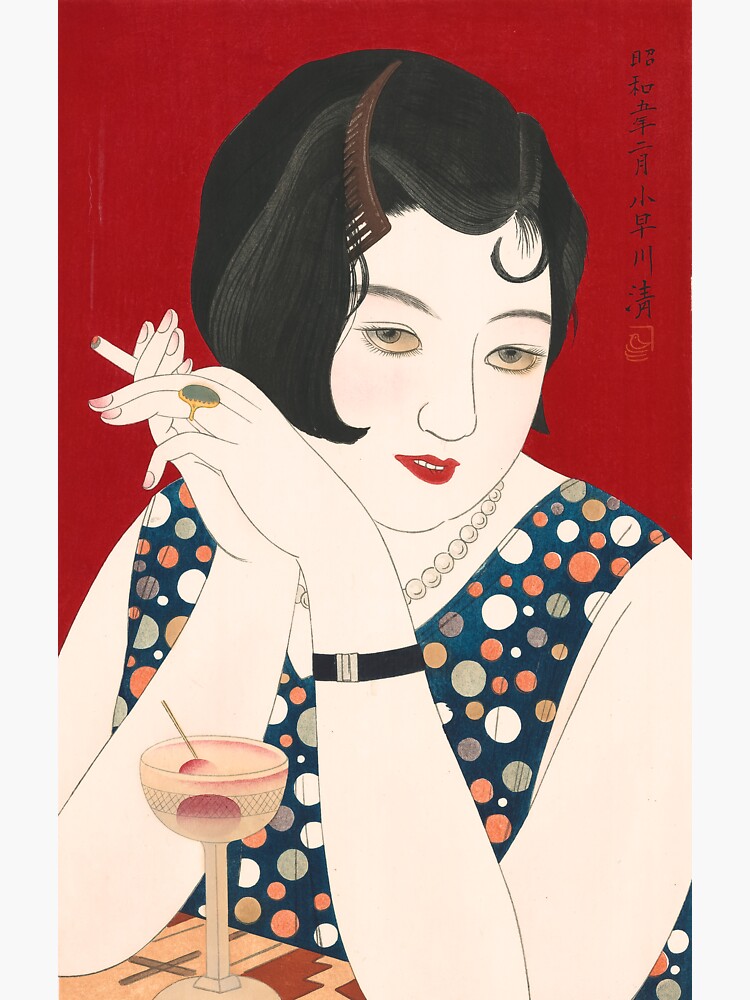This is a detailed illustration depicting an Asian woman, possibly Japanese, seated at a bar table with a cocktail. The art style resembles a painting or cartoon. She has short, cheek-length black hair and is adorned with a hair comb. The woman is facing the viewer, her face tilted downward slightly, and she is wearing red lipstick. Her fair skin contrasts with her cloudy, possibly intoxicated, hazel or green eyes. 

She is dressed in a sleeveless dark blue-green polka-dot blouse with multi-colored and variously sized dots. Around her neck is a white pearl necklace. Her left arm displays a black bracelet or watch with a silver clasp, while her fingers of the other hand hold a cigarette. A notable accessory is her green-jewelled ring, possibly an emerald set in gold.

The table in front of her features a martini glass with an olive and a toothpick. The entire backdrop of the image is a solid red, accentuated by Japanese text on the right side, adding to the cultural context of the scene.